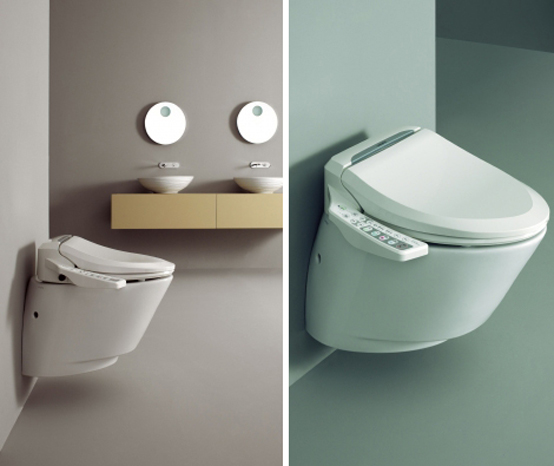The composite image features two vertically oriented, realistic photographs arranged to form a square. The left photo showcases an elegant, beige-toned bathroom with a sleek design. It includes a wooden countertop holding two modern, bowl sinks each topped with a round, glass mirror. Mounted on the wall to the left is a sophisticated, wall-mounted toilet with no back tank, harmoniously colored to match the beige decor and finished with a closed seat lid.

The right photo zooms in on the same wall-mounted toilet but in a bathroom with a greenish color scheme. The toilet here appears light green, blending with the environment, and is accompanied by a control panel brimming with numerous buttons, indicating advanced functionalities. The contrasting color palettes between the two bathrooms underscore their modern aesthetics, unified by the distinctive, innovative toilet design featured prominently in both images.